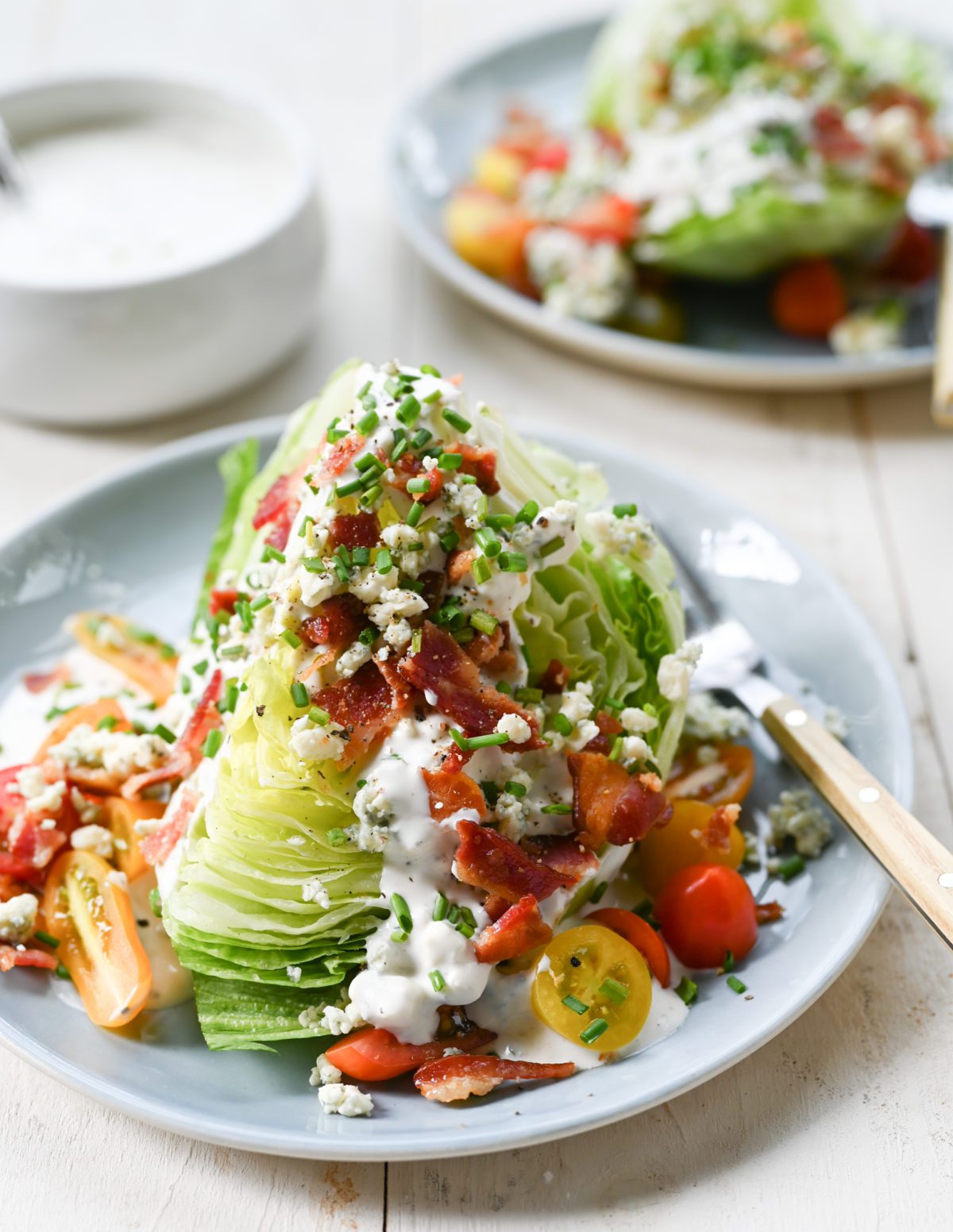The image captures a close-up of an artfully arranged salad, prominently displayed on a cream-colored plate sitting atop a white-painted wooden table. The salad comprises a generous mound of greens, accented by vibrant bell peppers, tomatoes, and crumbled cheese. In addition, it features toppings such as bacon, chives, onions, and both yellow and red baby tomatoes, some of which are cut in half. A distinct ranch dressing is drizzled over the salad, with a bowl filled with more dressing situated to the left. Adding to the composition is a fork, which rests on the plate. In the background, another similar salad dish appears blurred, hinting at a dining experience likely in a restaurant setting.